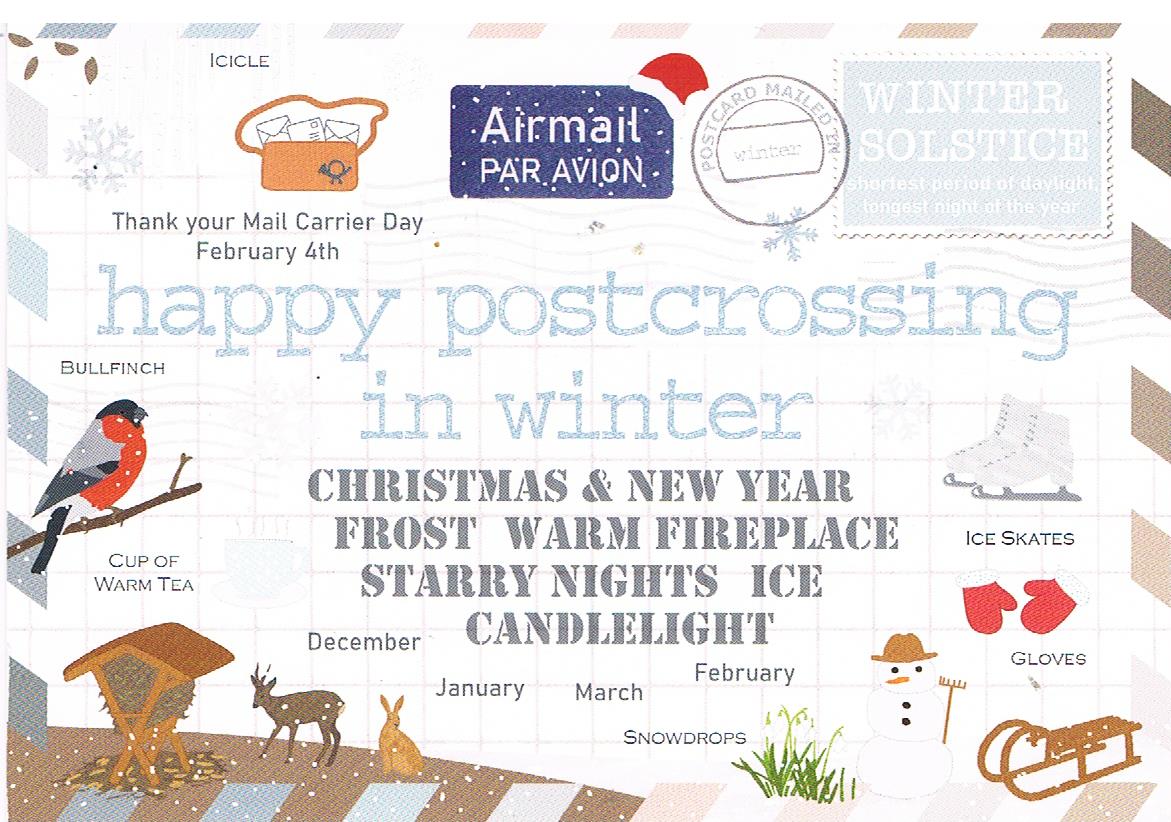This image depicts a festive, postcard-like flyer with a white background and pastel colors. It features a decorative striped border and numerous illustrations and text celebrating winter and the holiday season. In the top right corner is a mock postage stamp reading "Winter Solstice - Shortest period of daylight, longest night of the year," along with a "Mailed in Winter" postmark. To the left, there is an "Air Mail Par Avion" label, and just below, a note recognizing "Thank Your Mail Carrier Day, February 4th." Dominating the center in bold letters reads "Happy Postcrossing in Winter." Following this, smaller text lists phrases like "Christmas and New Year, frost, warm fireplace, starry nights, ice, candlelight," and the months "December, January, March, February."

The bottom section is crowded with various whimsical, clip-art-style images: a bullfinch perched on a branch labeled "bullfinch," a bird's nest beside a "cup of warm tea," a playful deer and bunny near "snowdrops," a snowman with a sled, red gloves, and a pair of ice skates. This charming visual captures the essence of winter festivities and joys, combining elements of postal traditions and seasonal cheer.